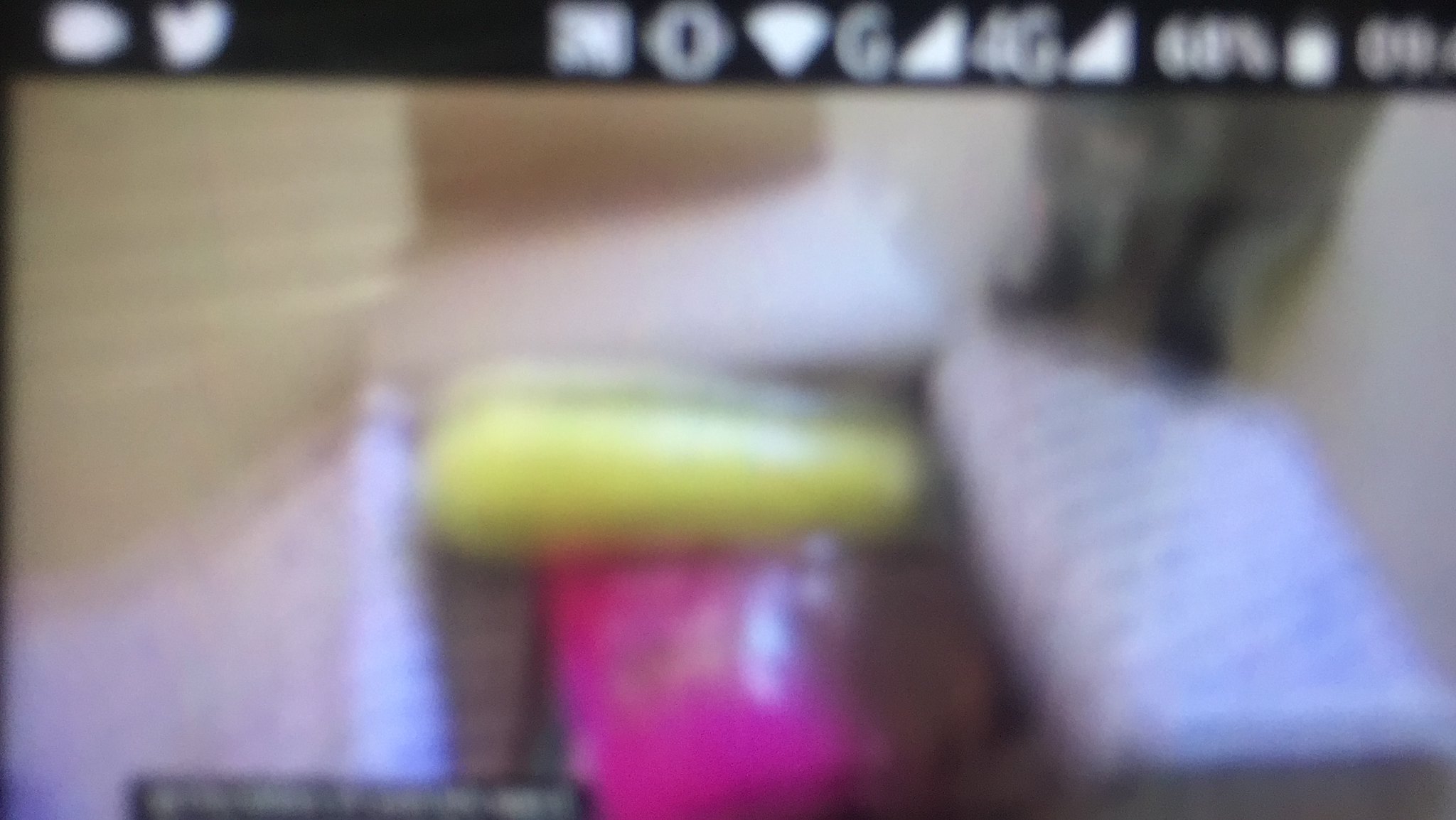A very blurry, rectangular color image likely taken as a screenshot. The image is horizontally oriented and difficult to decipher due to the poor quality. At the top left corner of the image, a few app icons are visible, although they are indistinct. One icon potentially resembles a Twitter bird, with another unidentified icon next to it. To the right of these icons, a series of status icons can be seen, including a '4G' network indicator, and what appears to be a battery percentage reading of either 64% or 68%. An additional 'G' character is present next to the '4G' symbol. The lower portion of the image contains a completely blurred-out scene featuring bright pink, yellow, and white colors. The indistinct shapes suggest it might depict objects like pillows or toys, but the details remain indiscernible.